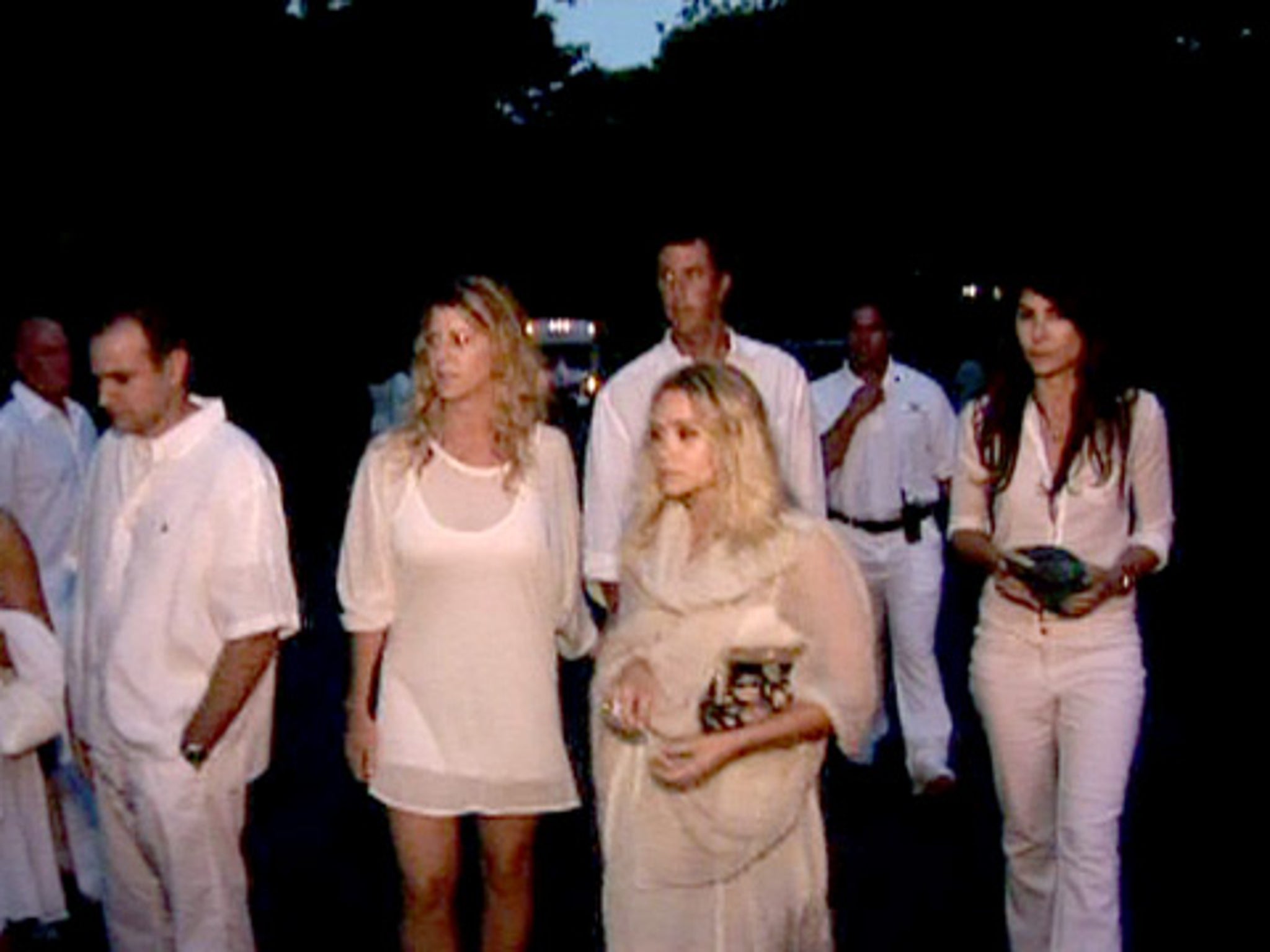This photograph, taken outside at night, features a group of mostly middle-aged Caucasian individuals. The scene is dimly lit, with the dark surroundings faintly revealing tree branches and a light blue sky peeking through at the top. The image captures eight people prominently in the foreground, all dressed in white or off-white attire, likely suggesting a themed gathering such as a white party. Despite the blurred and poor resolution, notable details include a dark-haired woman in a white shirt and pants on the left, a blonde woman in a short white dress next to another blonde woman similarly attired, and a dark-haired man in white shirt and pants to the right. A balding man in a buttoned-up white shirt and pants is also visible. In the far background, the illuminated front of a white bus or mode of transportation can be seen. The muted, orangish tones on the individuals’ faces hint at the age and quality of the photograph, with the camera's flash providing the primary light source.